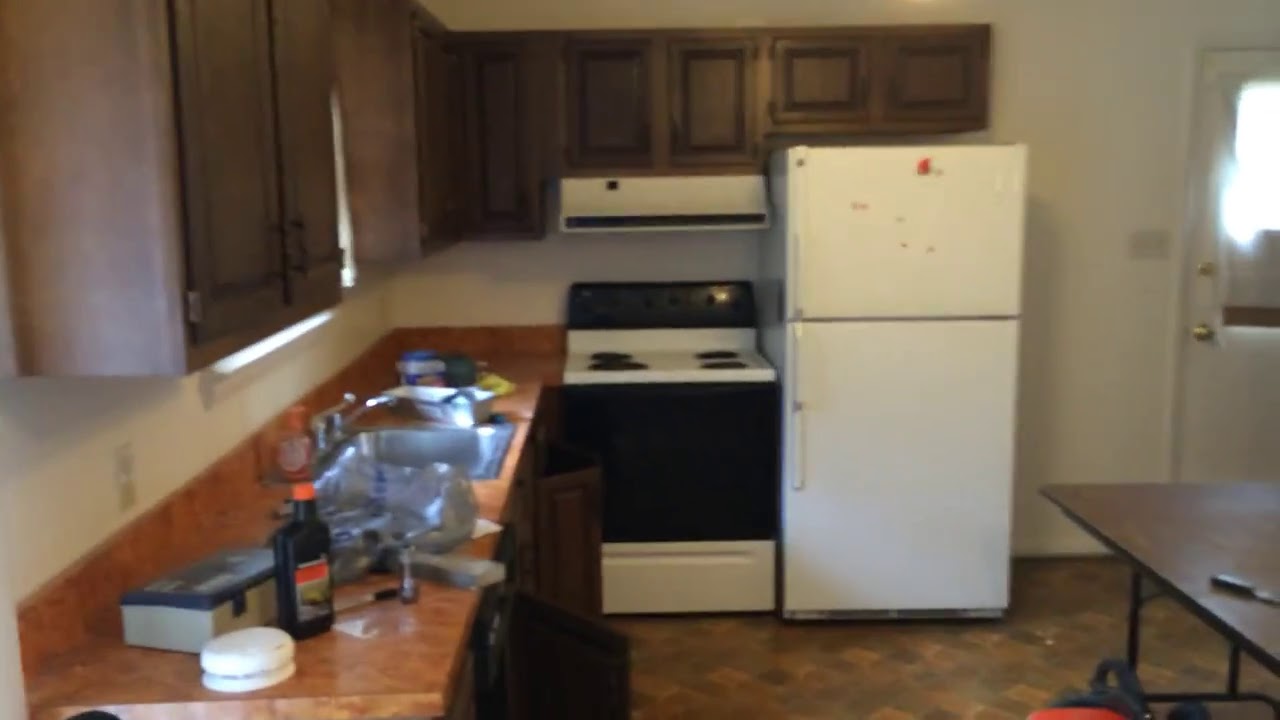The image depicts an old, run-down kitchen illuminated by sunlight streaming through a door in the top right corner. The floor features a small, rectangular wooden mosaic pattern in varying shades of dark and slightly lighter brown. In the center of the image, an antiquated white refrigerator stands beside an electric coil stove with a black front and a white hood. The kitchen is lined with dark brown wooden cabinets and an orange-tinted Formica countertop, which is cluttered with assorted tools, perhaps indicating ongoing plumbing work. Additional items such as a possible Drano bottle, smoke alarm, and soap can be spotted near the sink. This interior setting, showcasing white, brown, red, gray, tan, dark gray, blue, orange, and yellow hues, gives the impression of a mid-day scene in someone's personal kitchen amidst a renovation or repair.